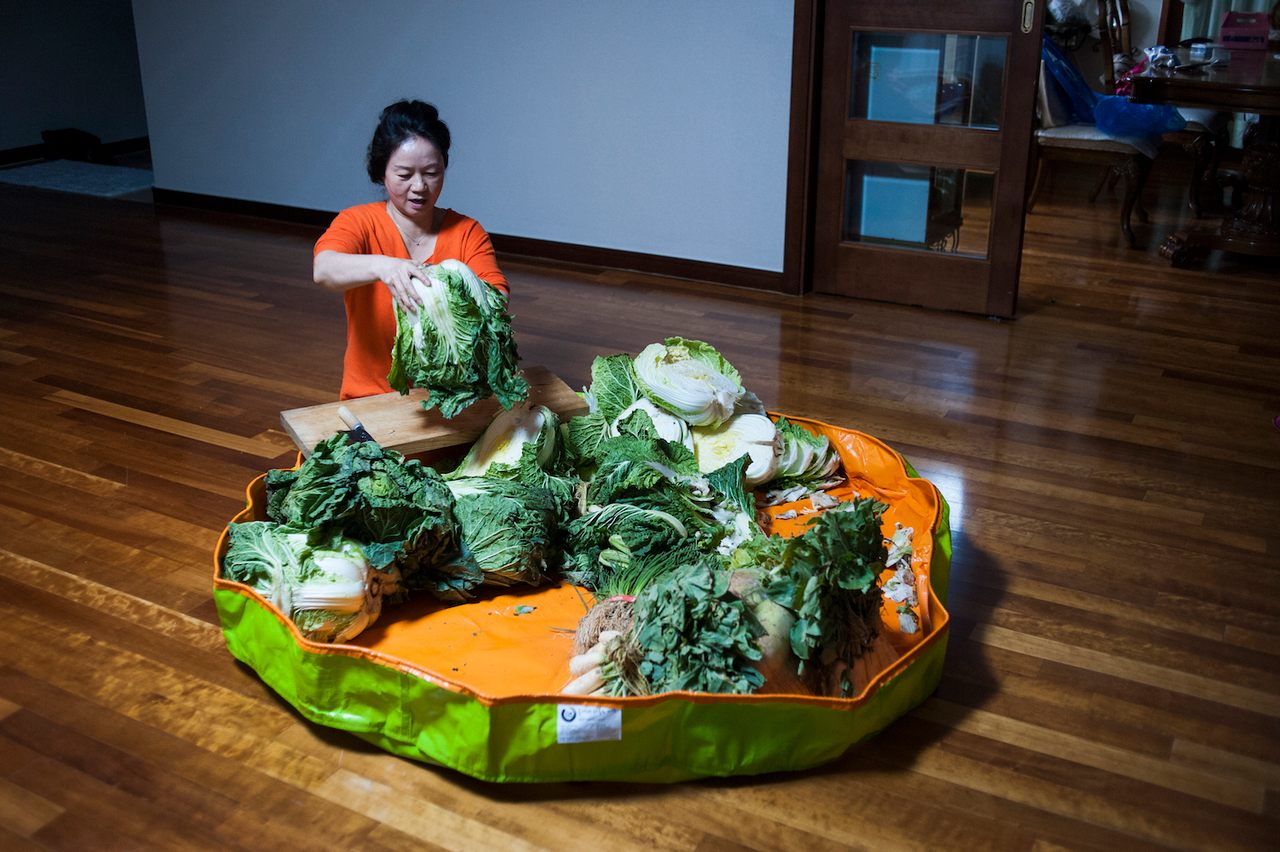This color photo features a Korean woman kneeling on the wooden floor of her open living room. The space, which has white walls and a sliding glass door leading to the kitchen, allows a glimpse into the adjacent dining area where a chair and a blue bag or jacket can be seen. The woman is identifiable as Asian, with her dark hair tied up, and is dressed in a bright orange short-sleeve t-shirt. In front of her, there is a large, soft kiddie pool with orange and yellow interiors filled with various vegetables, including heads of cabbage with deep green leaves, chives, and daikons. A wooden cutting board rests on top of the pool, and she is holding a head of cabbage over it, with a knife next to her. This setup suggests that she is in the process of preparing ingredients for making kimchi, a traditional Korean fermented cabbage dish.